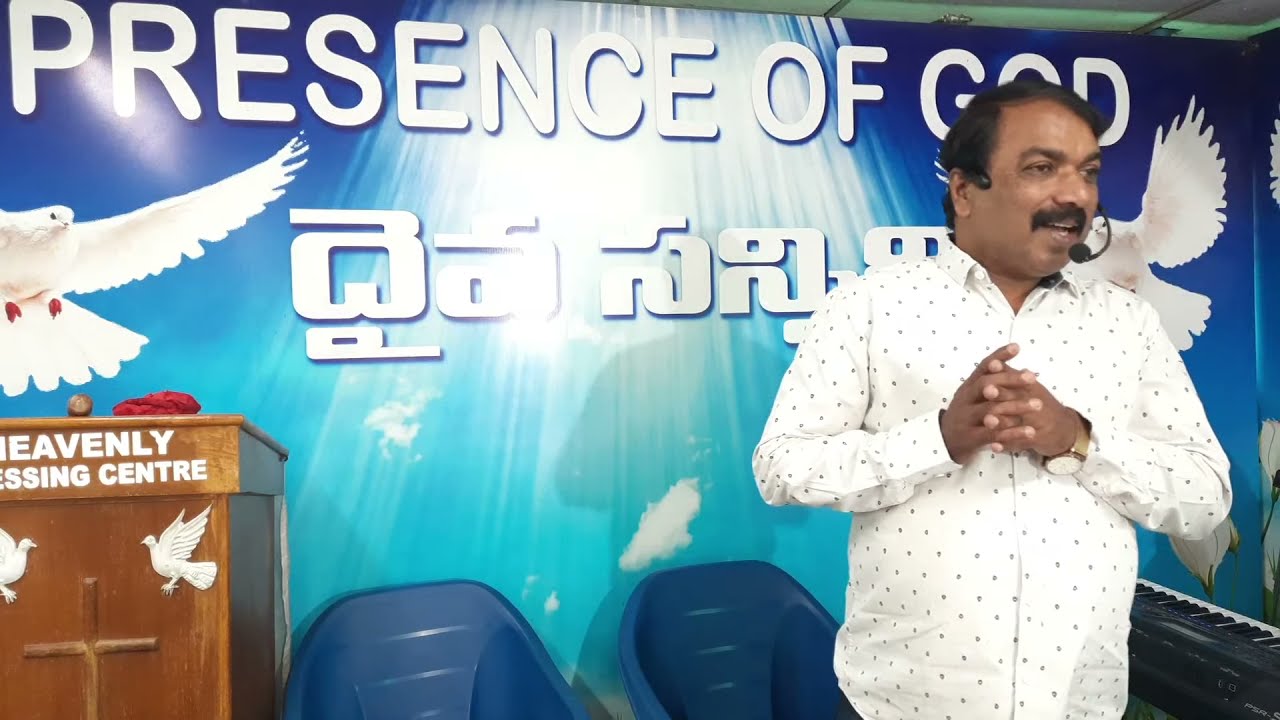A man with dark brown skin and a mustache stands with his fingers interwoven in front of his chest. He wears a white shirt adorned with gray dots and a gold watch on his right wrist. A microphone wraps around his head, positioned near the left side of his mouth. Behind him, a banner displays the words "PRESENCE OF GOD" in uppercase, followed by text in a foreign script, possibly Hindi or Arabic. White birds with outstretched wings decorate the banner. To his left, a wooden podium features a partially visible inscription: "Heavenly Blessing Centre." Two white doves and a cross are also visible on the podium. In the far-left corner, behind the man, stand two silver plastic chairs, and to his right, the keys of a keyboard are visible. The background hue is blue, adding a serene atmosphere to the scene.